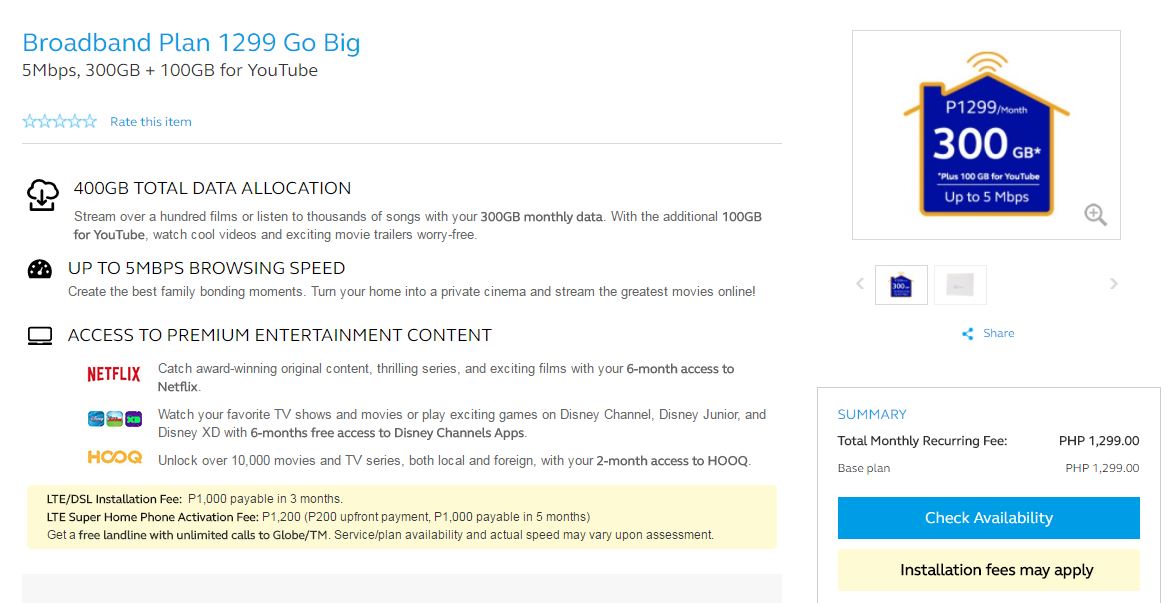On a predominantly white background webpage, the page header on the top left features bold cyan blue text stating "Broadband Plan 1299: Go Big". Directly beneath this, bold black text provides details: "5 Megabytes, 300 Gigabytes, 100 Gigabytes for YouTube". Below these details, there is a rating section displaying "0 out of 5 stars" accompanied by the prompt "Rate this item".

On the far right-hand side of the page, a small rectangular box with a thin black border features a dark blue house icon with an orange roof, outlined in orange and adorned with wireless signal bands. This box contains bold white text reading "P1299/month" and highlights "300 GB" in bold. Underneath, additional bold white text states, "plus 300 Gigabytes, 100 Gigabytes for YouTube, underline up to 5 Megabytes per second."

In the bottom right-hand corner, bold blue text reads "Summary" followed by black text detailing "Total Monthly Recurring Fee: PHP 1299," "Base Plan: PHP 1299." The section also includes a dark blue button with white text in the center that says "Check Availability." Next to this button is another light tan box with black text indicating, "Installation fees may apply."